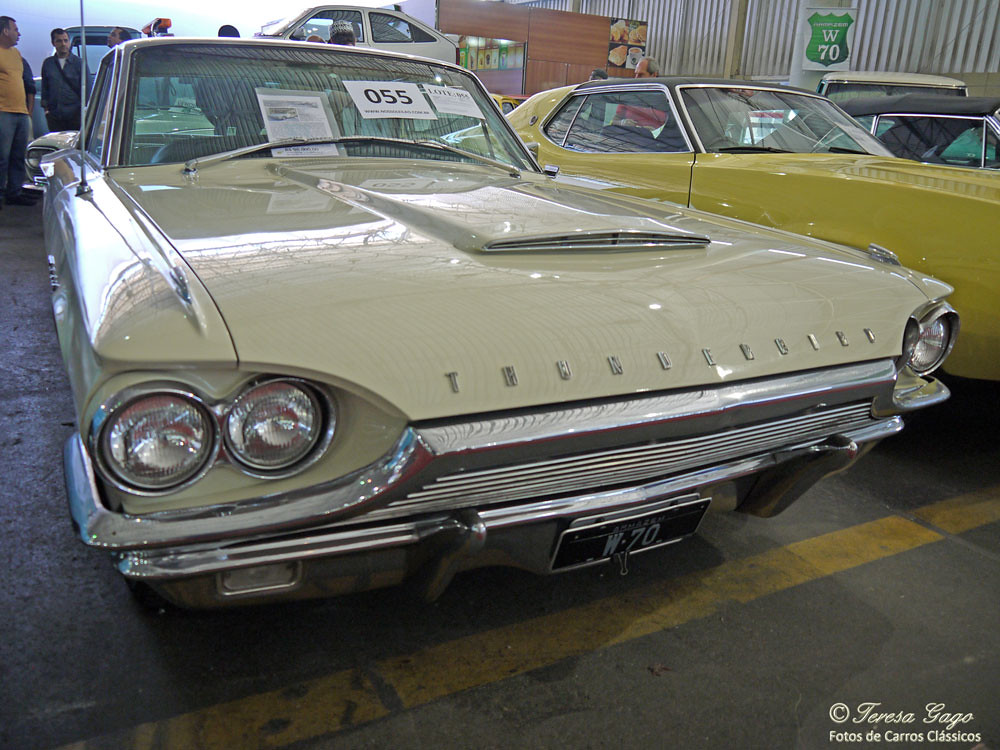The photograph captures a close-up view of the front of a classic Thunderbird car, prominently showcasing its faded cream-beige color and shiny, well-maintained exterior. The "THUNDERBIRD" name is clearly emblazoned in capital letters on the hood. The car features a distinctive air intake above the engine area. The license plate reads "W70," with white text on a black background. Several other classic cars, including a yellow one, are visible adjacent to the Thunderbird, indicating that the scene is set in a used car lot or a classic car gathering, marked by red and yellow parking lines. In the background, a group of people, dressed for mildly cold weather, are admiring the cars. Inside the window of the Thunderbird, white signs with black writing can be seen, possibly indicating car details or a sale listing. The photograph bears a watermark in the bottom right corner that reads "Teresa Gago. Fotos de Carros Clásicos," suggesting it was taken by a Spanish-speaking photographer.